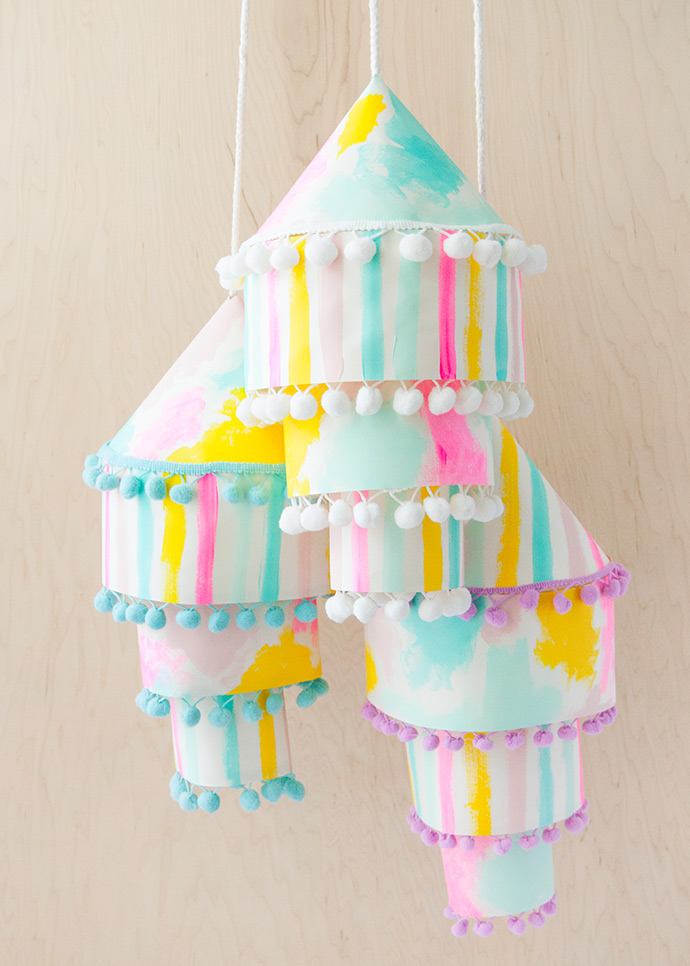The image depicts a handcrafted ceiling decoration against a pale birch plywood background. Hanging from the ceiling are three white strings, each supporting a colorful, circus tent-like lantern. These lanterns, which resemble an inverted three-layer cake or kites, are constructed from white fabric adorned with vibrant stripes and blotches of colors such as yellow, pale blue, aqua, pink, and lavender. Each lantern has a conical top similar to a child's birthday hat, but slightly broader. The cone is fringed with decorative pom-poms: white on the central lantern, blue on the left, and lavender on the right. Below the cone, each lantern has two successive, smaller bands of fabric, also adorned with matching pom-poms, creating a nested, tapering effect. The intricate details and playful colors lend a whimsical, circus-themed charm to the scene.